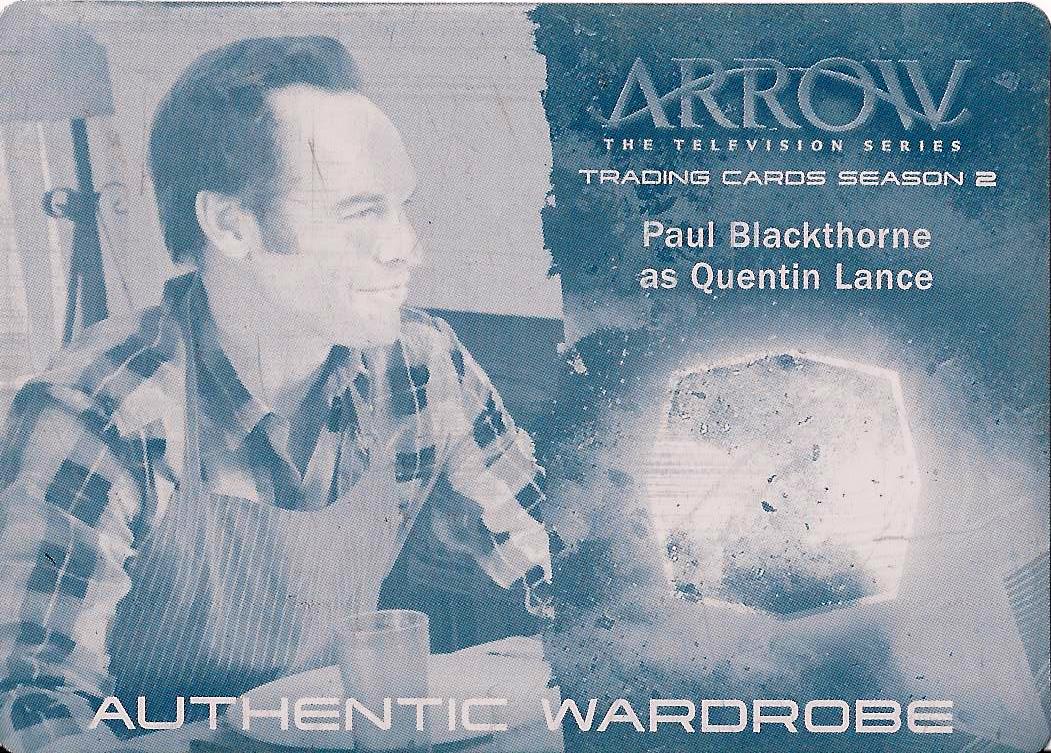The image resembles a vintage advertisement, characterized by faded blue and white colors with visible creases. On the left side, a Caucasian man with a slight smile is seated at a table. He has sideburns, wears a checkered shirt and a striped bib or apron, and has an empty plate and cup in front of him. Behind him are a wall and a lamp. The right side features an advertisement for "Arrow: The Television Series," styled as a front cover or trading card. The text, primarily in white against a dark blue background, reads: "Arrow" at the top, followed by "The Television Series," "Trading Card Season 2," "Paul Blackthorne as Quentin Lance," and at the bottom, "Authentic Wardrobe." A six-sided white gem-like image is also depicted beneath the names.